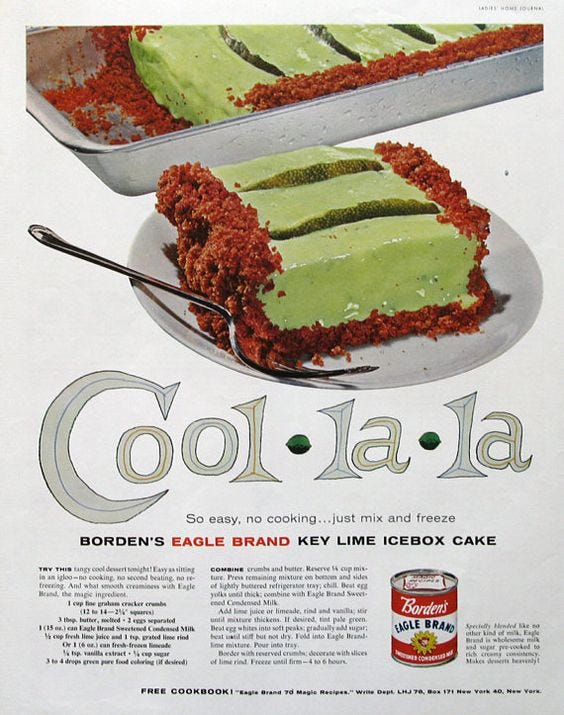This image appears to be a vintage magazine advertisement for Borden's Eagle Brand Key Lime Icebox Cake. The ad is set against an all-white background and features a silver rectangular tray at the top filled with a green cake, which is actually a Key Lime Icebox Cake. The surface of the cake is green, and it has a red crust, made from graham cracker crumbs as per the recipe. The cake is somewhat glossy in appearance, and a slice has been cut out revealing its creamy texture. 

Below the tray, there is a separate white plate with a slice of the cake and a silver fork, highlighting the individual serving. The text under the image reads "Cool la la! So easy, no cooking, just mix and freeze." Further below, it promotes the product: "Borden's Eagle Brand Key Lime Icebox Cake." A can of Borden's Eagle Brand, recognizable by its distinctive red and white label with a cow graphic, is featured prominently. Additional text appears to be a detailed recipe, though it is too small to read clearly in the image. The advertisement emphasizes the convenience of preparing the cake, making it an appealing summer dessert option.